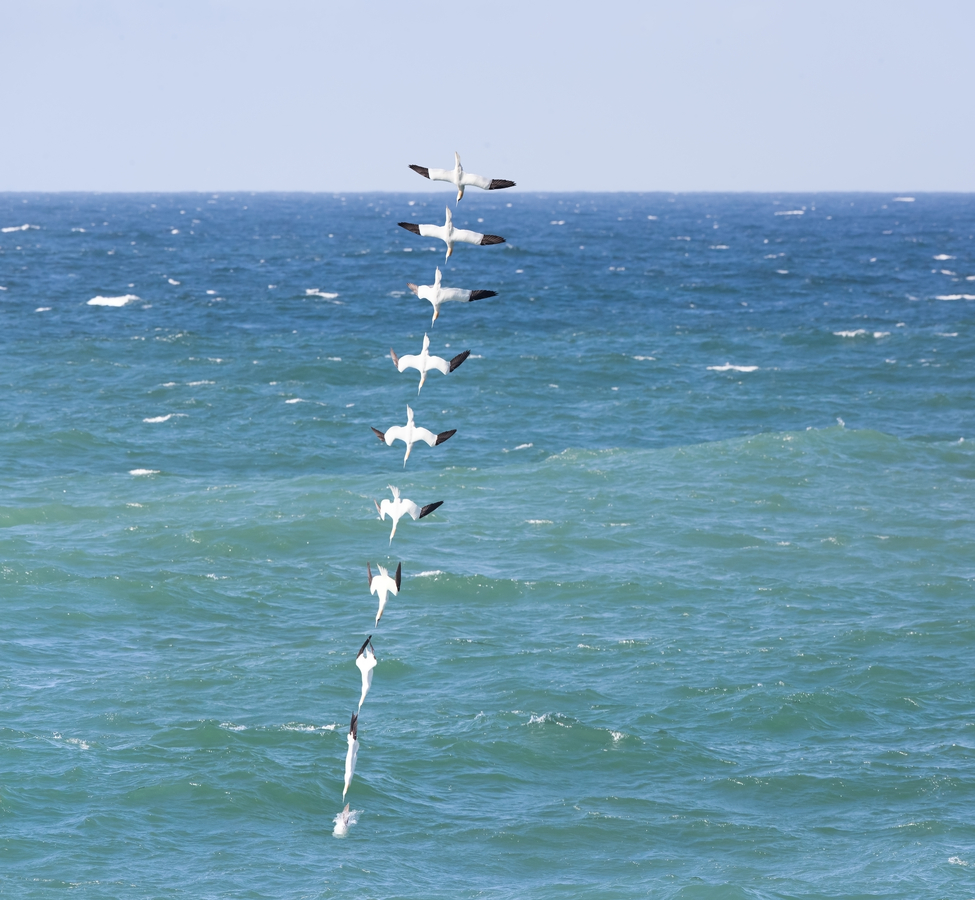This captivating square photograph, taken during the daytime, depicts the serene ocean with turquoise, green, and blue hues mixed with white-capped waves. The sky above is a clear, light blue without any clouds. At the center of the image, a time-lapse composite shows a white bird with black-tipped wings, reminiscent of a cormorant or seagull, diving into the water. There are ten distinct frames of the bird, captured in quick succession and overlaid vertically, illustrating its graceful dive. Starting just above the horizon with its wings fully extended, the bird gradually pulls its wings in, forming an arrow shape by the second-to-last frame. In the final frame, the bird is almost completely submerged, having pierced the calm ocean's surface in a precise, downward trajectory that slightly veers to the left. This detailed composite masterfully captures the essence and motion of the bird's elegant descent into the water.